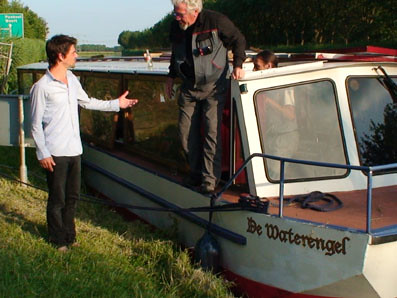The image is a small, detailed photo taken outdoors during the daytime, showing a scene by a canal or river. The rectangular image, around two inches tall by three inches wide, requires close inspection. Dominating the scene is a long boat named "De Waterengel," painted white with a blue stripe and brown text. The boat's front features a blue metal barrier and a reflective windshield. 

An older man wearing a long-sleeve black and gray jacket and gray pants is standing on the boat's ledge, looking down. He is reaching towards a younger man of Caucasian descent with short brown hair, barefoot and wearing a white button-up shirt and black pants, who is standing on the grassy embankment. The young man extends his left hand upward to assist the older man in disembarking.

Another individual, possibly wearing a white and gray short-sleeved shirt, is partially visible behind the older man, indicated by the top of their head. The grassy area contrasts with the dark, flat-topped boat, likely enclosed. In the background, beyond a hedge, a green street sign and trees flank the canal, adding to the tranquil outdoor setting.